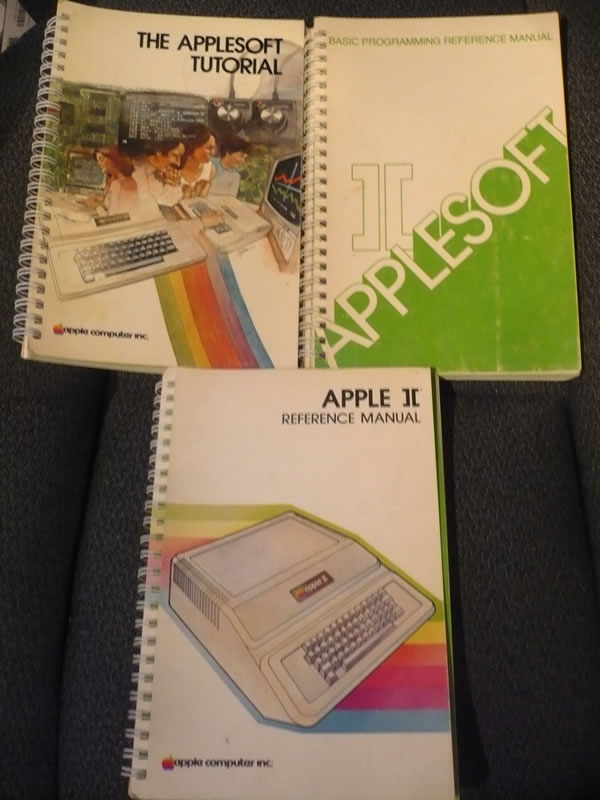This vertically oriented, multi-color photograph captures three spiral-bound booklets, which are staged on a dark gray chair cushion. The background is a muted blue, possibly the chair's upholstery. The booklets are arrayed with two on the top and one on the bottom. 

The top-left booklet, titled "AppleSoft Tutorial," shows a family using a large computer monitor and keyboard. A rainbow lines the monitor’s base, extending downwards. Its cover features a black typeface and an Apple Computer Inc. logo at the bottom left.

The top-right booklet, labeled "AppleSoft 2," has a white upper half with green text, and a green lower half. The Roman numeral "II" and text "Basic Programming Reference Manual" are prominently displayed. 

The bottom booklet, titled "Apple II Reference Manual," is primarily white and features an old Apple computer, represented by a keyboard with a square computer unit on top. A rainbow design arcs from the back to the front of the device, and the title is written in black font. A crease in the cushion's surface runs up the left side of the image, accentuating the arranged, nostalgic presentation of these vintage Apple manuals.